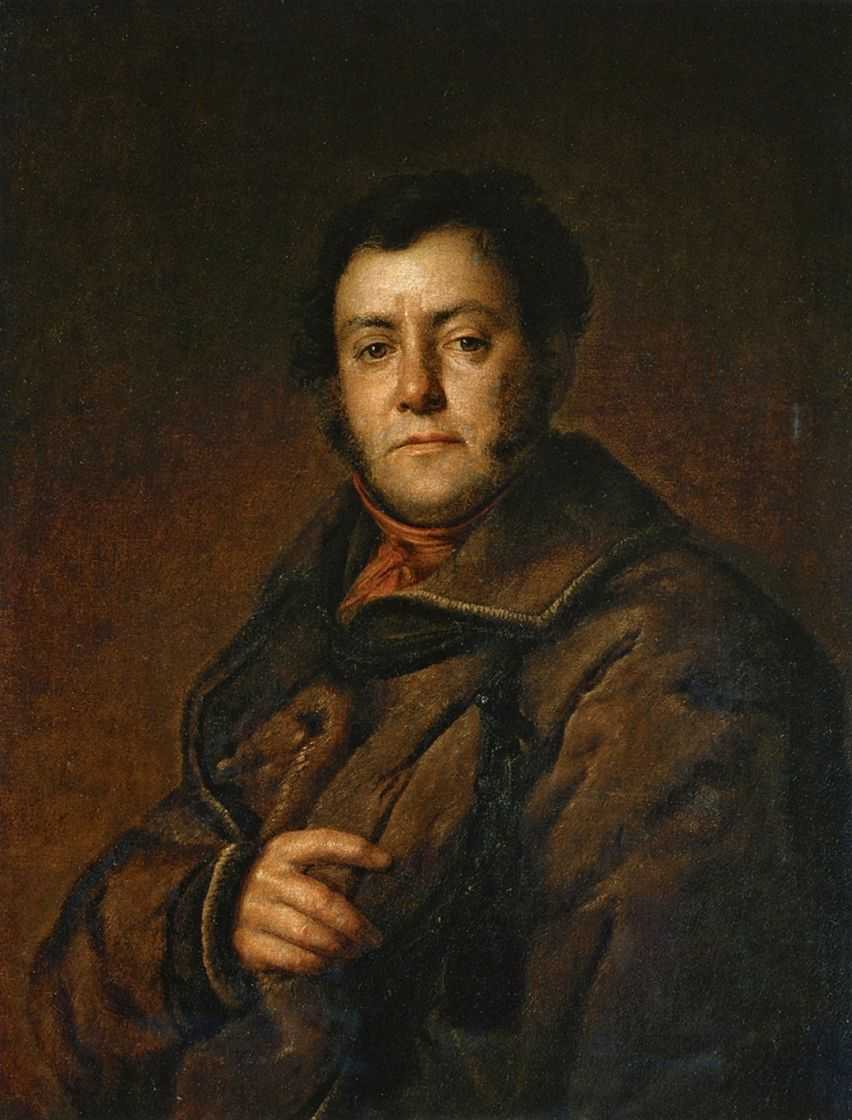This detailed oil painting is a formal self-portrait of a Caucasian man, approximately 30 years old, rendered in a style reminiscent of the 18th century. The background is predominantly brown with darker hues at the top, creating a somber atmosphere. The man, with his short, dark brown hair and distinctive mutton-chop sideburns that extend down to his jawline, has white skin and dark eyes. He is not smiling, imparting a serious expression on his face.

He is attired in a large, dark brown overcoat, hefty and seemingly adorned with gold and black braiding. The coat's fabric appears thick and heavy, further emphasized by its substantial collar. Beneath the overcoat, barely visible, the man is wearing a reddish-orange cravat or scarf, tied snugly around his neck. This garment adds a slight touch of color and intricacy to his otherwise muted attire. His right arm is extended outward, allowing his hand to be seen, while his left arm rests by his side, suggesting a formal and composed stance.

His attire, mannerisms, and the choice of colors used in the painting all contribute to a palpable sense of formality and historical grandeur, making the portrait an evocative representation of an era long past.